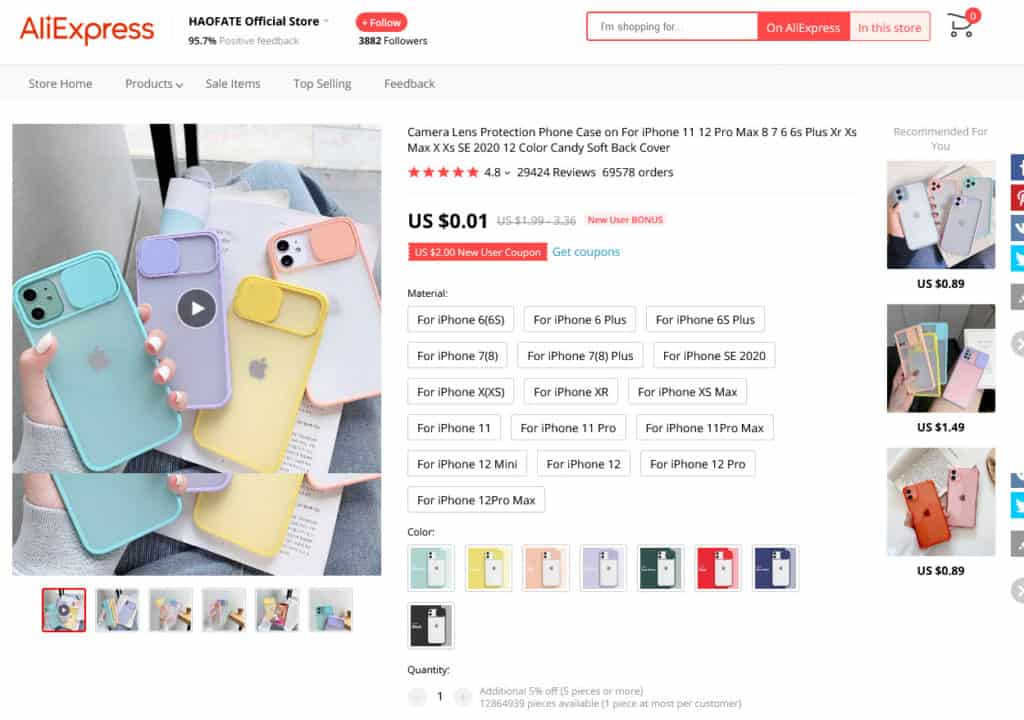This screenshot from AliExpress displays a product listing for a "Camera Lens Protection Phone Case" compatible with various iPhone models, including iPhone 11, 12, Pro Max, 8, 7, 6, 6S, Plus, XR, XS, Max, X, XS, SE (2020). The AliExpress logo in orange is positioned at the top left corner of the page.

In the main section of the page, the product title is centered above a prominently displayed image of four phone cases in teal, purple, yellow, and an orange-peach color. Directly below the title, the product has received a rating of 4.8 stars, as indicated by the star icons and numerical rating to their right. The price of the phone case is listed as US $0.01.

Below the price, there are options to select the suitable phone model, with each model being listed. Further down, there are color options available for the phone case, including teal, yellow, peach, lilac, green, red, blue, and black. 

To the right side of the page, there are images of alternative phone case options, each with individual pricing details beneath them. Additionally, there are sharing options for social media platforms such as Facebook, Pinterest, and Twitter, along with a copy link option. Some sharing icons are unclear, but the layout suggests a range of social sharing functionalities.

In summary, this detailed image depicts a comprehensive and user-friendly product listing for a versatile and colorful phone case on AliExpress.